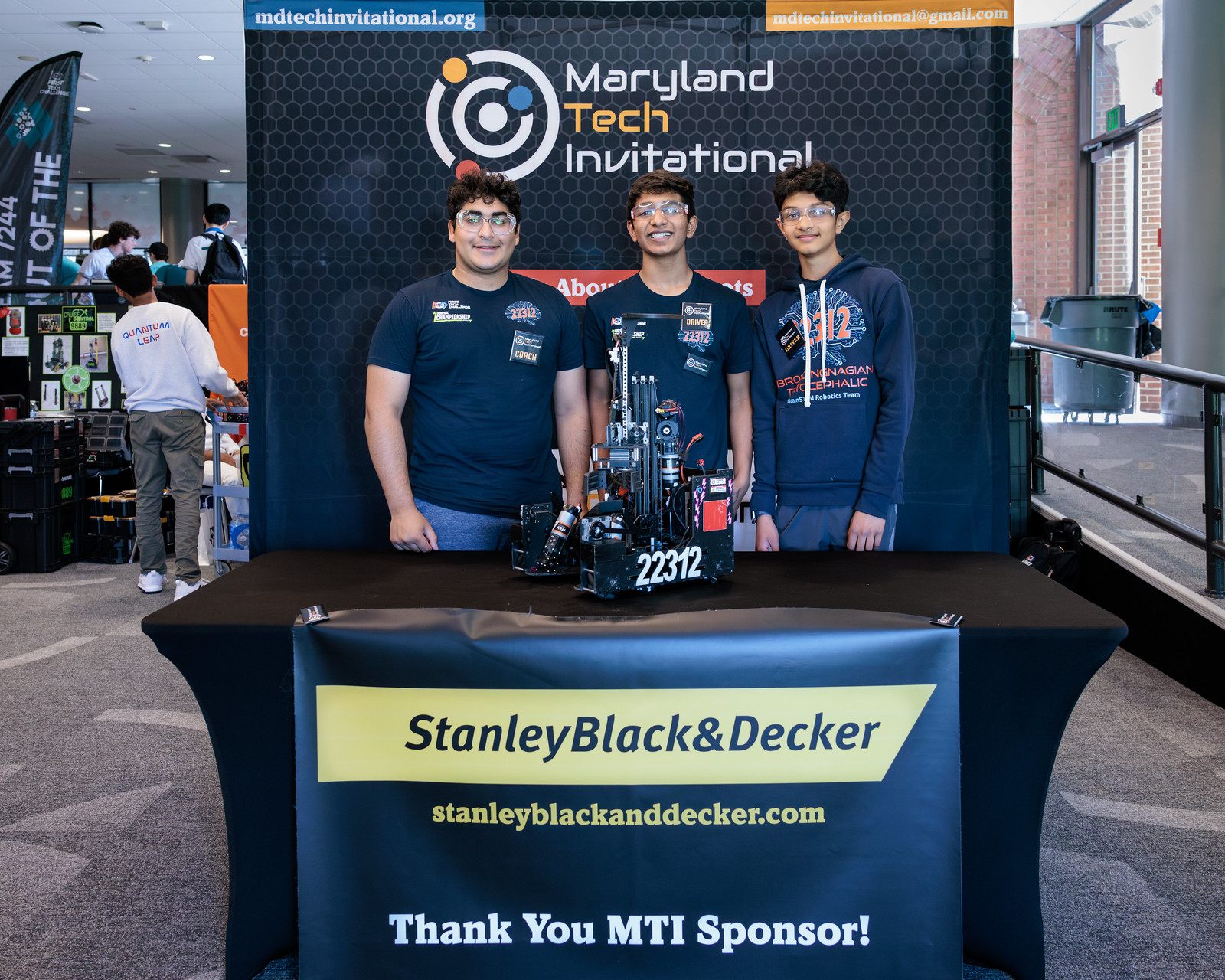This image features three young men, all in their early 20s, standing behind a table at what appears to be the Maryland Tech Invitational. They are positioned in front of a blue-navy banner adorned with circular designs and the event's logo, which resembles a rotating atom with blue, red, and yellow balls. The banner prominently displays "Maryland Tech Invitational" in white and gold lettering, along with the URL MDTechInvitation.org, and mentions Stanley Black & Decker as a sponsor.

The three men, each sporting safety glasses, short brown hair, and jeans, are dressed in blue attire. Two of them are wearing blue t-shirts, while the third is in a blue hoodie. Each shirt features tags and logos, including a distinctive sticker with the number 22312. They are standing beside a complex robotic unit, which also bears the number 22312 in white lettering.

Behind them, the indoor setting reveals a carpeted floor, people milling in the background, a ramp, and a trash can leading to a glass doorway. The display table in front of them is covered in a black cloth that showcases the text "Stanley Black & Decker" and the website StanleyBlackanddecker.com, followed by "Thank you, MTI sponsor."